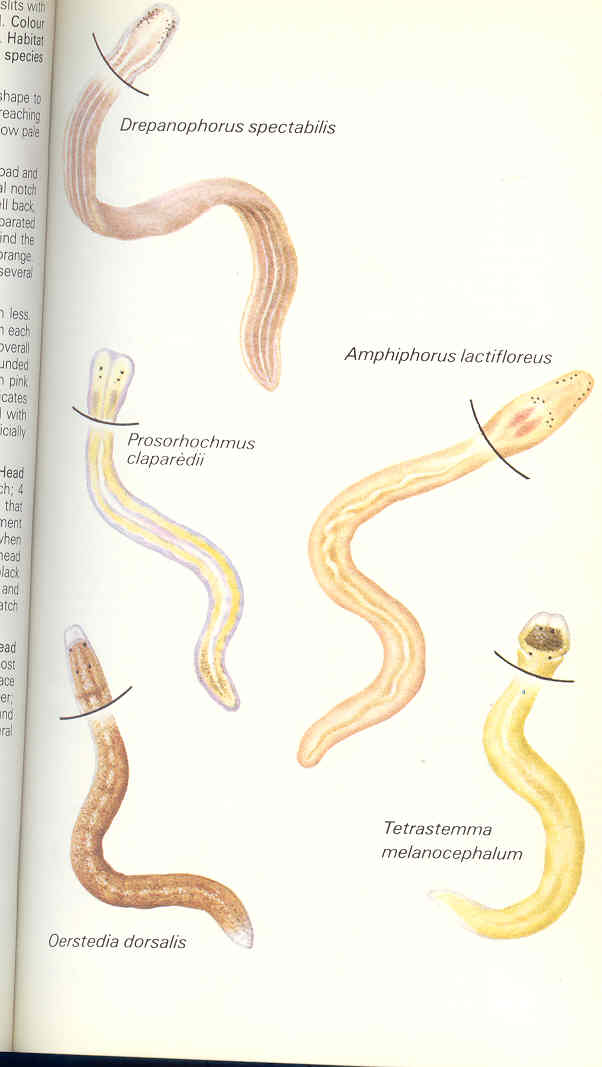This detailed scientific illustration from a textbook depicts various worm-like creatures, showcasing specific areas for head removal. At the top left corner is the brown Drepaniophorus spectabilis. To its right, a long, light orange worm is identified as Amphiphorus lactiflorus. Farther down, there's the yellow Prosorhochmus claparedii with distinct head sections. In the bottom left corner lies the brown Orstedia dorsalis. Lastly, the bottom right corner features the smaller, yellow Tetrastemma melanocephalum, characterized by its brownish head. Each worm is meticulously labeled, with clear indications of where to sever the head, enhancing the anatomical study of these diverse species.